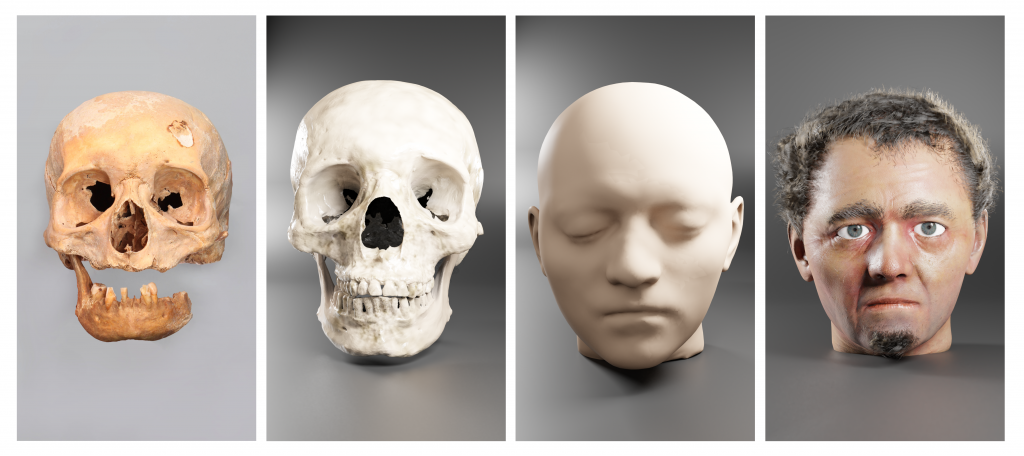The image is a compilation of four stages of a forensic facial reconstruction. The first section features a light tan skull, aged and damaged with a missing left mandible, several absent teeth, a cracked and dusty nose area, and right eye socket partially filled, potentially indicating a cause of death from a dent on the right side. The second section showcases the same skull but in a white, repaired state with a restored jaw, representing a complete skeletal head. The third section displays a smooth, monochromatic white bust with closed eyes and no hair, signifying a preliminary facial mold. The final section presents a detailed and lifelike representation of a man with short brown hair, hazel eyes, a small goatee, gray eyebrows, and slightly red lips, showing the reconstructed appearance of the skull's original owner. The background in all images is a consistent gradient of gray, adding to the clinical, scientific atmosphere of the reconstruction process.